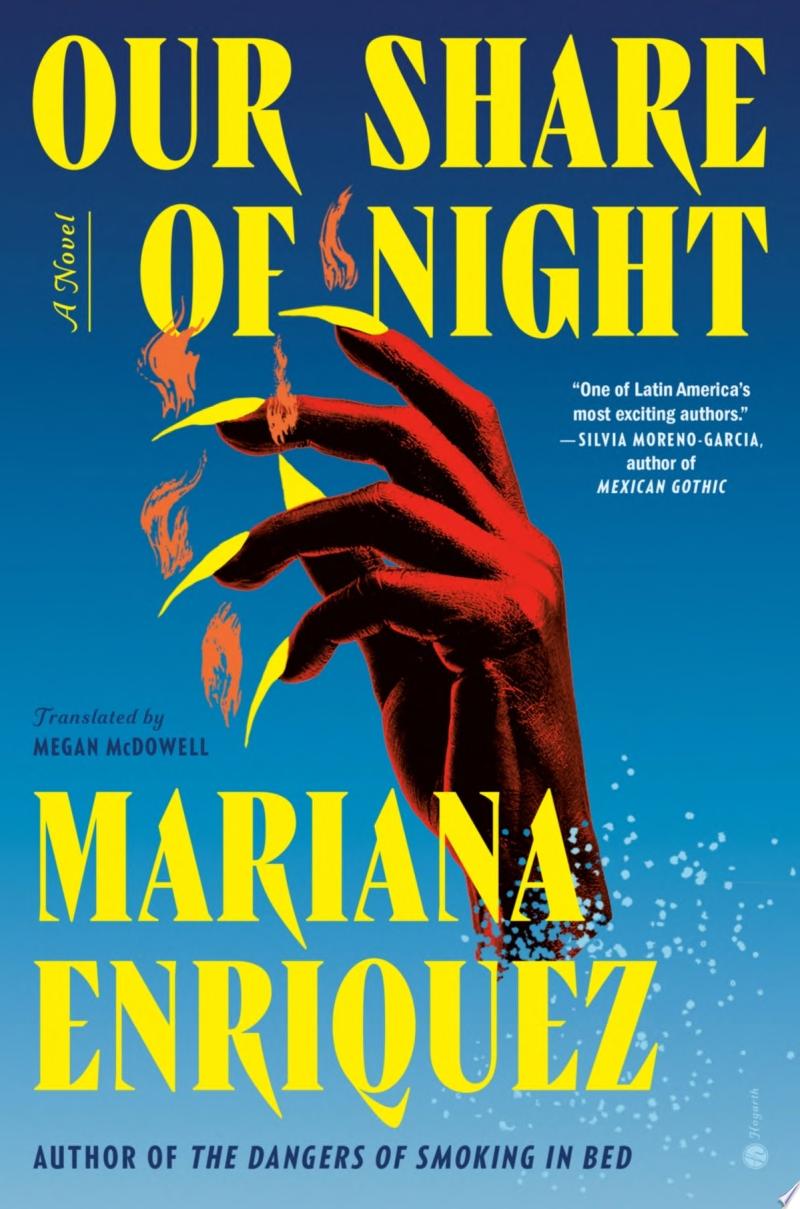The book cover features a captivating blue background with a gradient that lightens towards the bottom into a subtle light blue, accentuated by bubble-like patterns. Dominating the midsection of the cover is an illustration of a red hand, resembling a claw or a devil's hand, with long, menacing yellow nails. Extending from each nail are vivid orange flames. At the top, in bold yellow capital letters, is the title "Our Share of Night," with a tiny label indicating it is "A Novel." The bottom section showcases the author's name, Mariana Enriquez, in prominent text, followed by a smaller line that reads "Author of The Dangers of Smoking in Bed." Beneath this, it is noted that the book was translated by Megan McDowell. Additionally, a white text blurb lauds the author, Sylvia Moreno-Garcia, calling Enriquez "one of Latin America's most exciting authors."